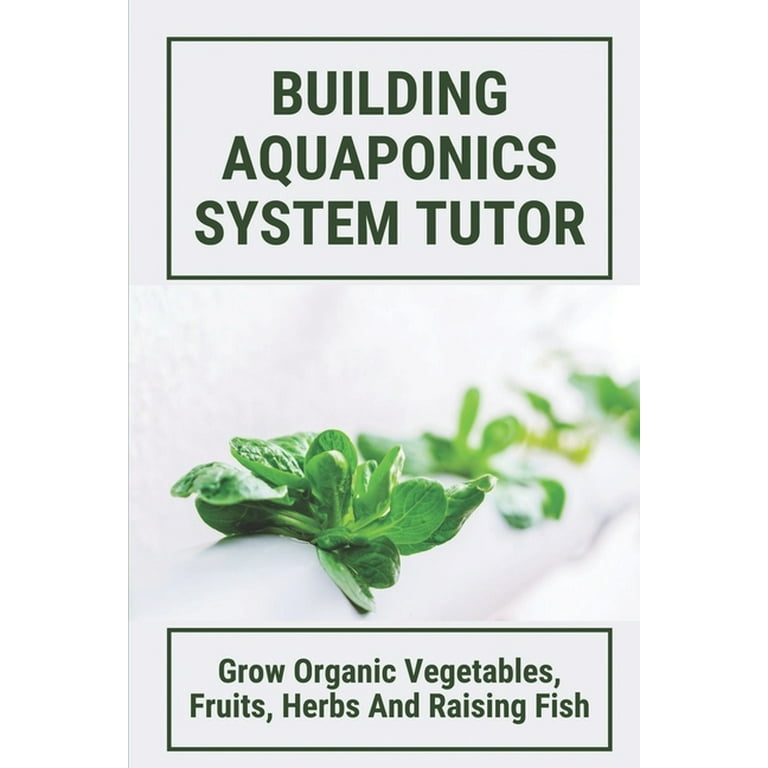The cover of a pamphlet, possibly a promotional material for an aquaponics system, features a predominantly white background. At the top, inside a black-bordered text box, the words "BUILDING AQUAPONICS SYSTEM TUTOR" are boldly printed in all caps, emphasizing the title. Central to the design is an image of a green leaf, possibly spinach or lettuce, prominently displayed in the foreground with fainter, blurred copies of the leaf fading into the background. Midway down the cover, there is an impression of green vegetation, hinting at the growth facilitated by the system. At the bottom, enclosed in a similarly thin black-bordered box, the text reads "Grow Organic Vegetables, Fruits, Herbs, and Raising Fish," explaining the benefits of the aquaponics system. The overall design combines elements of clarity and detail to illustrate the efficiency and productivity of this innovative gardening method.